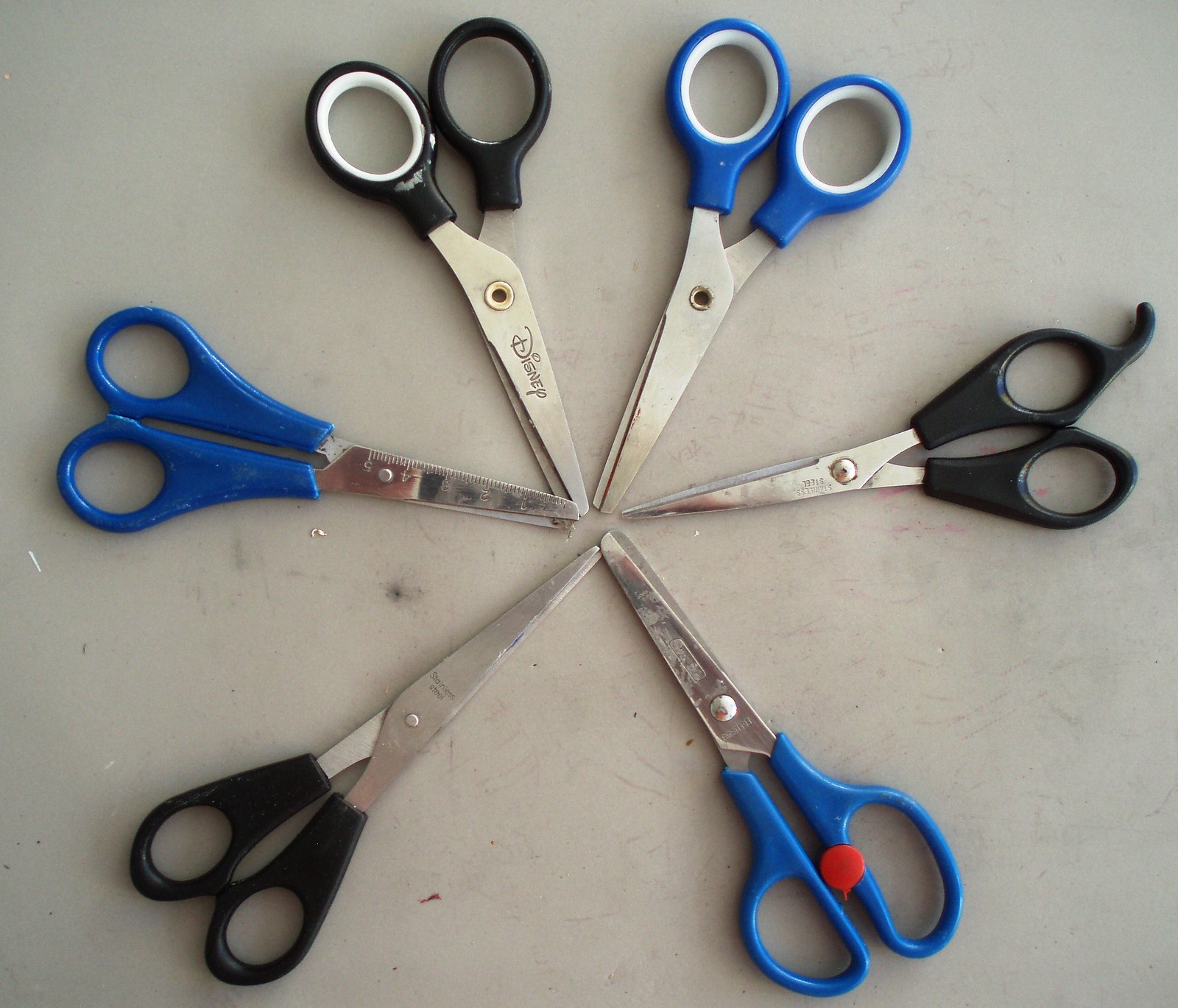The image is a slightly horizontally rectangular or square photograph depicting six pairs of scissors neatly arranged on a gray, somewhat scuffed-up surface, possibly a table or floor. The scissors are configured in a precise star or asterisk pattern with their stainless steel blades meeting at the center. Each pair features plastic handles: three in blue and three in black. Notably, the pair of black-handled scissors in the top left corner has "Disney" etched into the blade, along with a distinctive white circle in one of the handle holes. The handles alternate in color around the pattern, creating a visually balanced effect. The gray background, marked with some loose black scuffs, enhances the symmetrical arrangement of the scissors, with approximate blade lengths of four inches each.